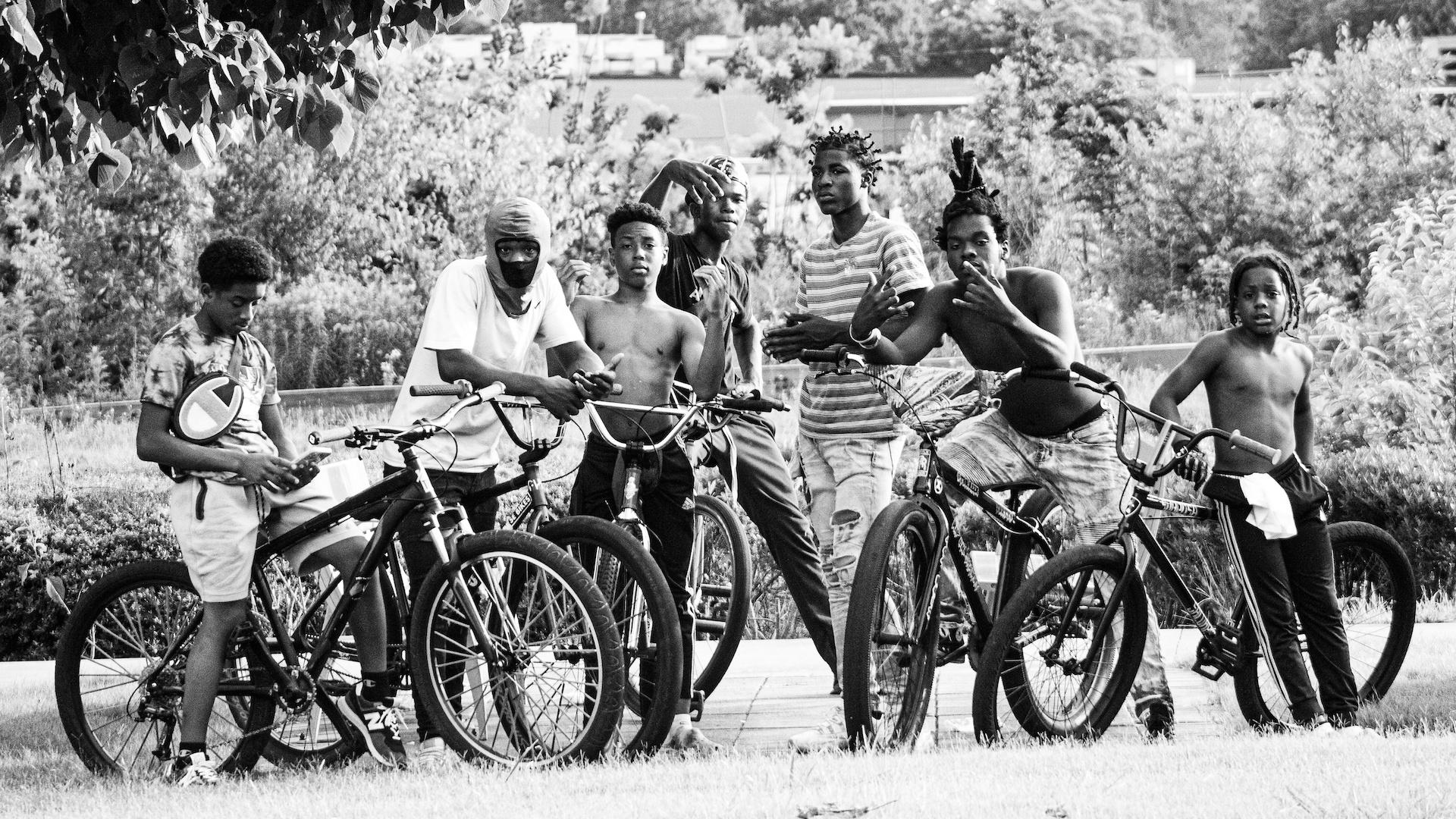This black and white photograph depicts a group of seven young Black boys in a park setting, enveloped by a background featuring dense trees, foliage, and a partially visible building peeking above a small fence. In the foreground, six boys are astride bicycles while one stands at the center. Differing in attire, some boys wear shirts while others are shirtless; a few sport shorts and others pants. 

From left to right:
- The leftmost boy is looking down at a phone.
- The second boy from the left has a mask covering his face, leaving only his eyes visible.
- The third boy, shirtless and wearing black pants, gazes directly at the camera.
- The central figure, standing without a bike, dons ripped jeans and a striped shirt, with hands folded as if in prayer.
- Next to him, a shirtless boy with hair standing up points his fingers downwards in a gesture.
- To his right is a boy, possibly the youngest, who leans on his bike with a white towel hanging from his pants, also showing a gesture akin to the “I love you” sign in sign language.
- The rightmost boy, although not explicitly described, fits the collective context of this casual yet poignant ensemble. 

The varied attire and activities, combined with the natural backdrop, give the image a dynamic and vibrant youthfulness, framed by the timeless contrast of black, white, and shades of gray.